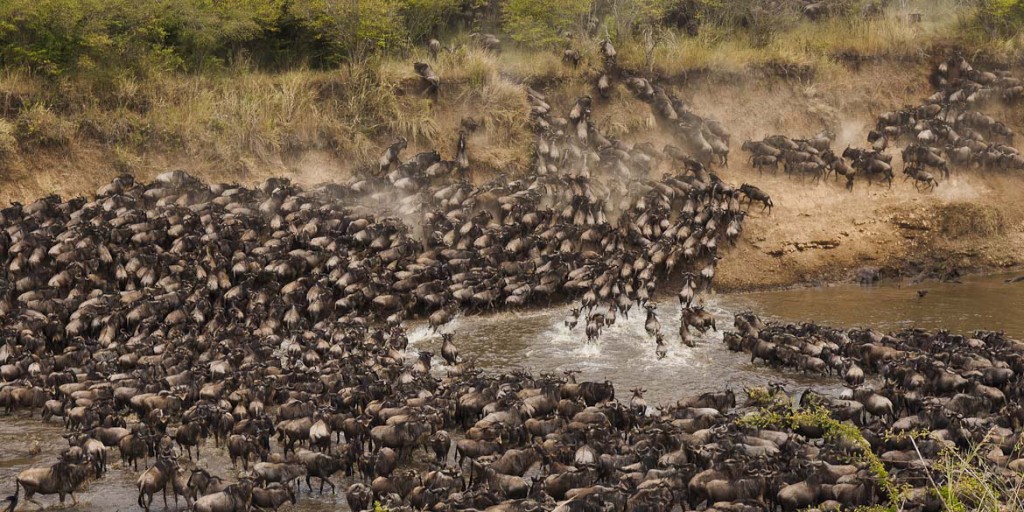In the image, a large herd of brown buffalo is depicted congregating around and within a river or lake, forming an upside-down question mark shape. The scene features a wide variety of animals, predominantly buffalo, all walking on four legs, some standing on the dry, lightly grassed terrain at the water's edge, while others wade through or drink from the water. The backdrop includes patches of gray dry brush with some green foliage seen from the bottom right to the top left of the foreground. In the background, a few cowboys can be discerned herding the animals, adding to the image's overall sense of motion and purpose as the animals peacefully travel together towards the embankment on the other side of the water.